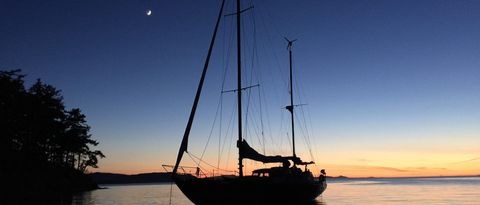The image depicts a serene evening scene featuring a large sailboat silhouetted against a calm sea. The sky transitions from a deep blue at the top to a lighter blue and then a yellowish-orange hue near the ocean's horizon, indicating either just before sunrise or just after sunset. In the top left corner, a crescent moon glows faintly against the darkening sky. The sailboat, situated centrally, has two tall poles and a thin mast with numerous wires extending from top to bottom. On the right side of the boat, a fabric roof is visible. To the bottom left of the image, there's a dense cluster of tall trees, suggesting the proximity of an island or shore. The overall image has a horizontal orientation, being more than twice as wide as it is tall. The sea reflects a calm, almost grayish surface, adding to the tranquil atmosphere of the scene.